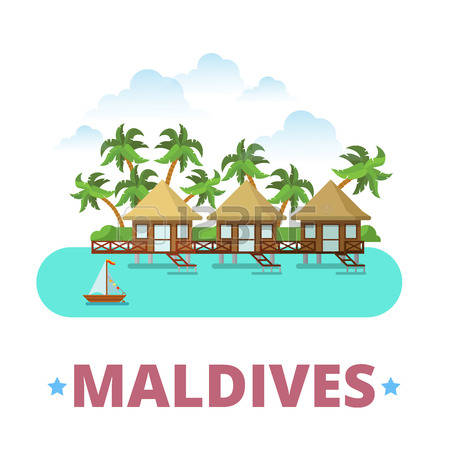In this colorful cartoon-style computer graphic, an inviting scene of the Maldives is depicted. Against a backdrop of light blue water and a white sky accentuated with fluffy clouds, three small wooden cabanas stand on platforms. Each cabana, brown with white doors and yellowish, pyramid-like roofs, rests on a pier-like structure surrounded by water. In the foreground, a red sailboat with white sails and a little reddish flag is sailing past these quaint huts. Behind the cabanas, lush greenery including large palm trees and green bushes enhances the tropical setting. At the bottom of the image, the word "MALDIVES" is displayed in pink capital letters, flanked by blue five-pointed stars, establishing the exotic locale.